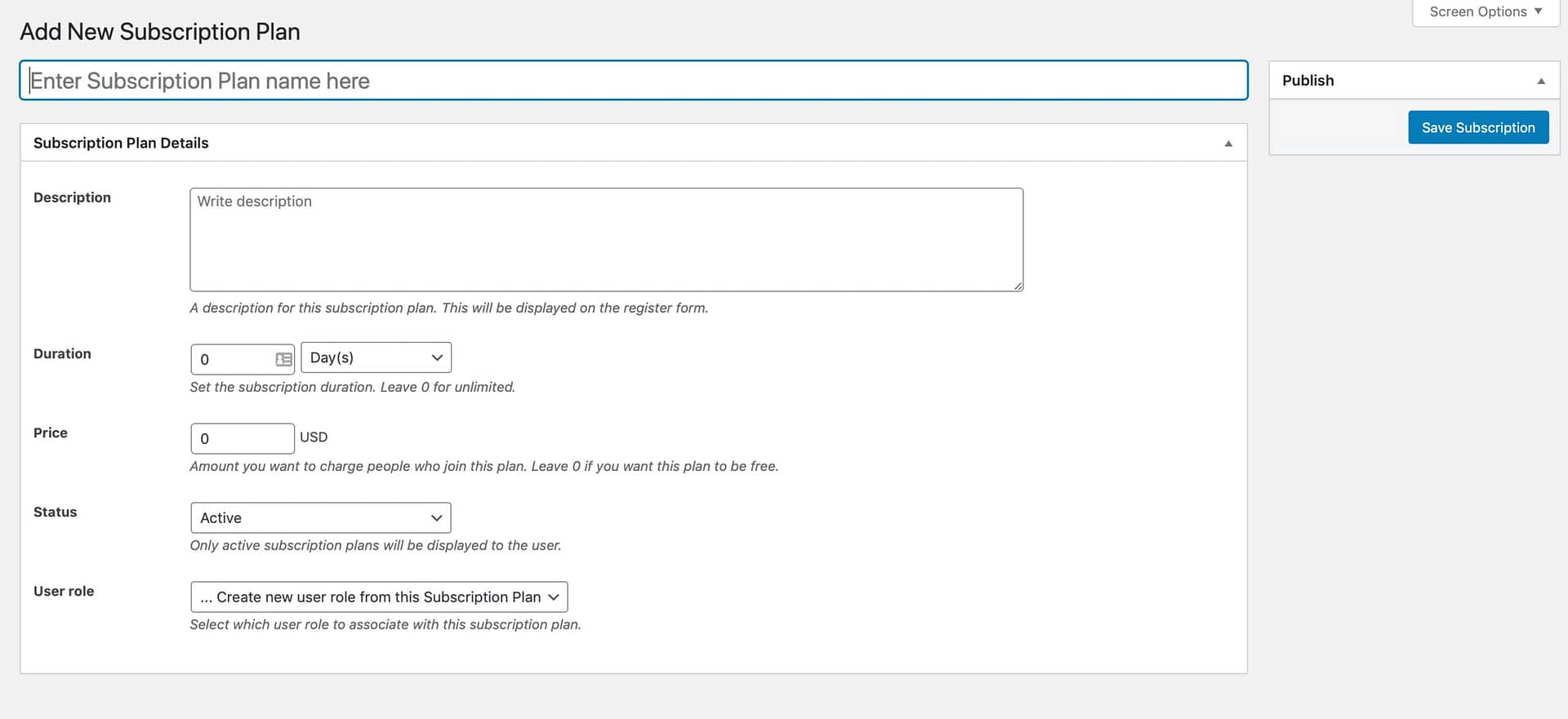The image depicts the "Add New Subscription Plan" interface. At the top left corner, "Add New Subscription Plan" is prominently displayed. The background of the interface is gray. Below the title, there is a white text input bar that nearly spans to the right but remains centered with the bottom section.

On the right side, there is a vertical menu composed of two items: "Publish," with an up arrow icon to its right, and a "Save Subscription" box located just below the "Publish" bar. On the left-hand side, a large white section titled "Subscription Plan Details" is visible. Beneath this, there is a "Description" label followed by a larger text input box for entering the details. Below the description box, there is a line for specifying the "Duration" in days. 

Following the duration field, there is a "Price" section for entering the subscription cost. Below the price section is a "Status" section, likely for indicating whether the plan is active or inactive. Finally, at the bottom, there is a "User Role" section for assigning user roles related to the subscription plan.